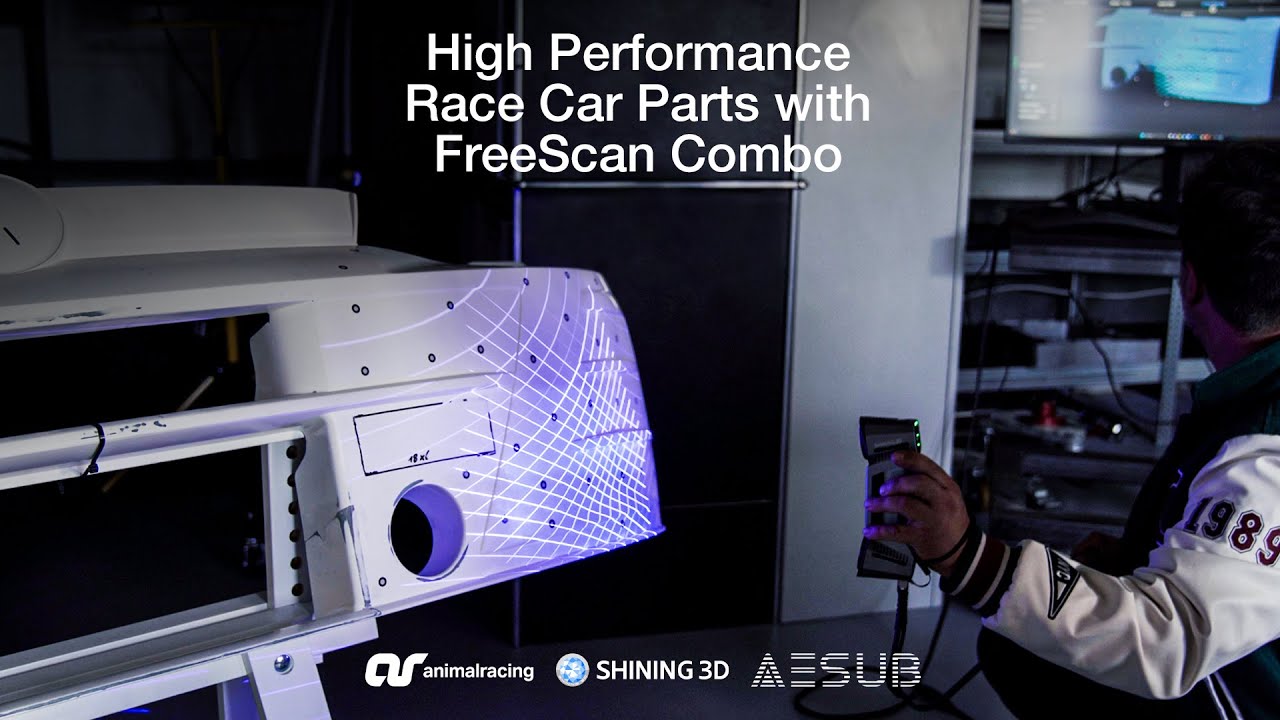A detailed color photograph advertises high-tech racing technology within an indoor setting filled with electronic equipment. The most prominent feature of the image is a person standing on the right side, wearing a letterman's jacket with "1989" emblazoned on the left shoulder. They are holding a sophisticated scanning device, although the specifics of the technology are advanced and somewhat unclear. Their attention is directed towards a computer monitor in the background, which displays what they are scanning. Below this monitor, a tangle of wires and various devices can be seen.

Central to the image is a glowing purplish-white box, likely the object being scanned. The upper section of the photograph contains text in white lettering that reads, "High Performance Race Car Parts with Free Scan Combo." At the bottom of the image, the brands "Animal Racing," "Shining 3D," and "AESUB" are prominently displayed, marking the collaborative effort behind this advanced technology. The overall composition suggests an advertisement centered on cutting-edge automotive components and scanning solutions.